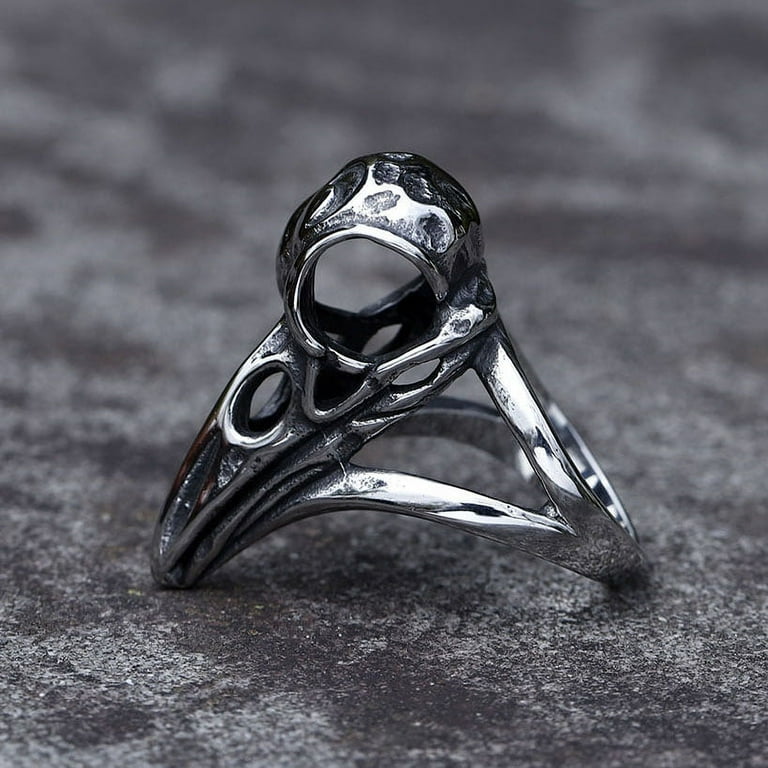The black and white macro photograph depicts a small, shiny metal object with a complex design, which is presumably a part of a ring, bracelet, or some form of jewelry. The object is lying on a textured, gray surface that resembles cement or tar, adding a rough contrast to the smooth, silver sheen of the metal. The main structure of the object is triangular, featuring a conspicuous oval or circular opening at the top that faces outward, much like the eye-hole of a historic witch doctor mask. The metal has varying shades of gray, with darker areas suggesting slight tarnishing or shadows. Despite its intricate design, the exact purpose or classification of the object remains ambiguous, lending it an intriguing and somewhat mysterious aura.